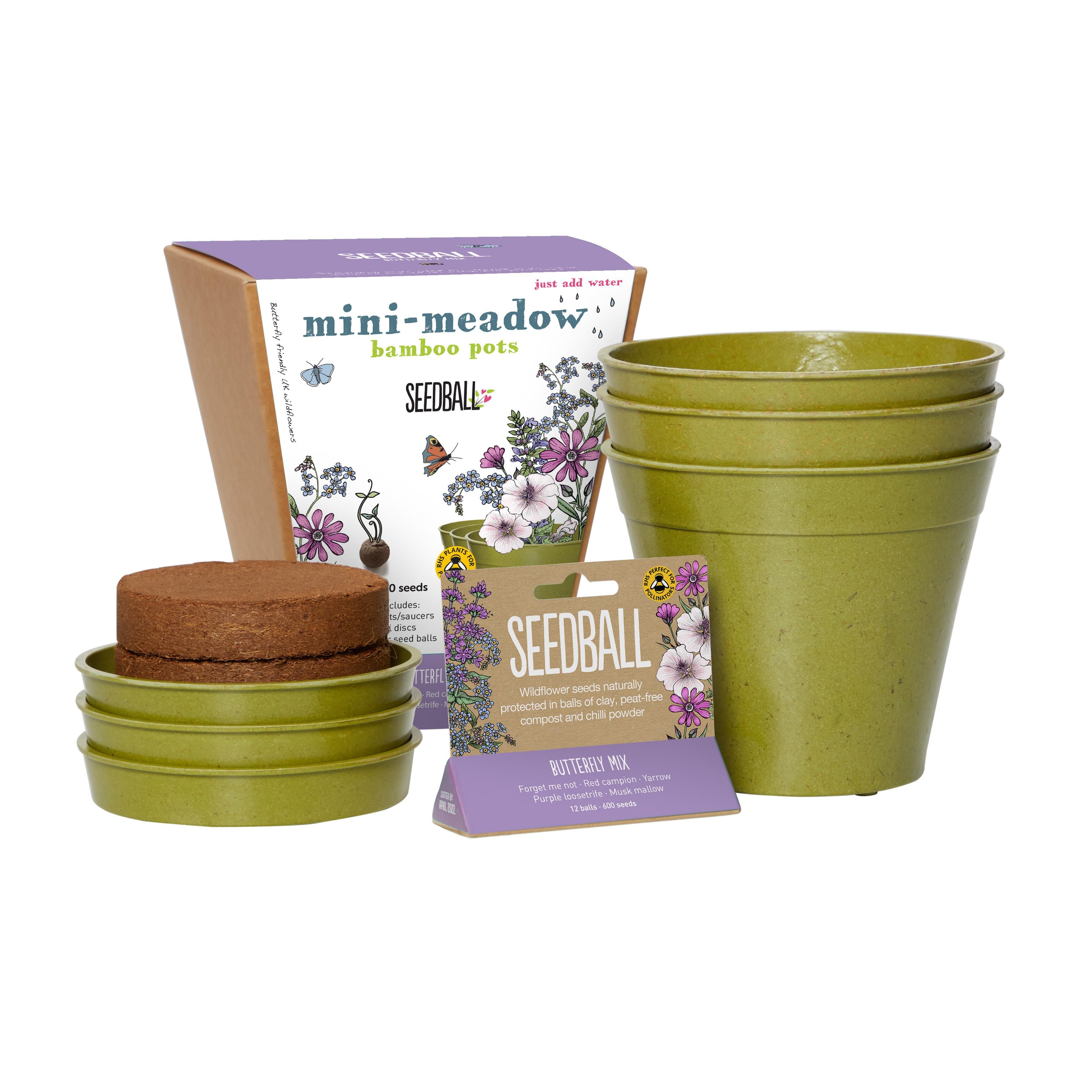The image showcases a detailed product arrangement of a home planting kit against a white background. At the forefront are three olive green planter bases accompanied by shallow dishes of the same color, serving as drainage bases. Inside these dishes are brown compressed soil disks, likely made from cocoa liner. Centrally positioned in the image is a package with a purple top, labeled "Mini Meadow Bamboo Pots Seed Ball - Just Add Water." This package features illustrations of pink flowers and a monarch butterfly. Next to it, there is a plaque stating, "Seed Ball, Wildflower Seeds Naturally Protected in Balls of Clay, Peat-Free Compost, and Chili Powder." The seed mix includes varieties such as Butterfly Mix, Forget Me Not, Red Campion, Yarrow, Purple Loosestrife, and Musk Mallow, containing 12 balls with a total of 600 seeds. This comprehensive kit allows buyers to create mini meadows effortlessly by just adding water.